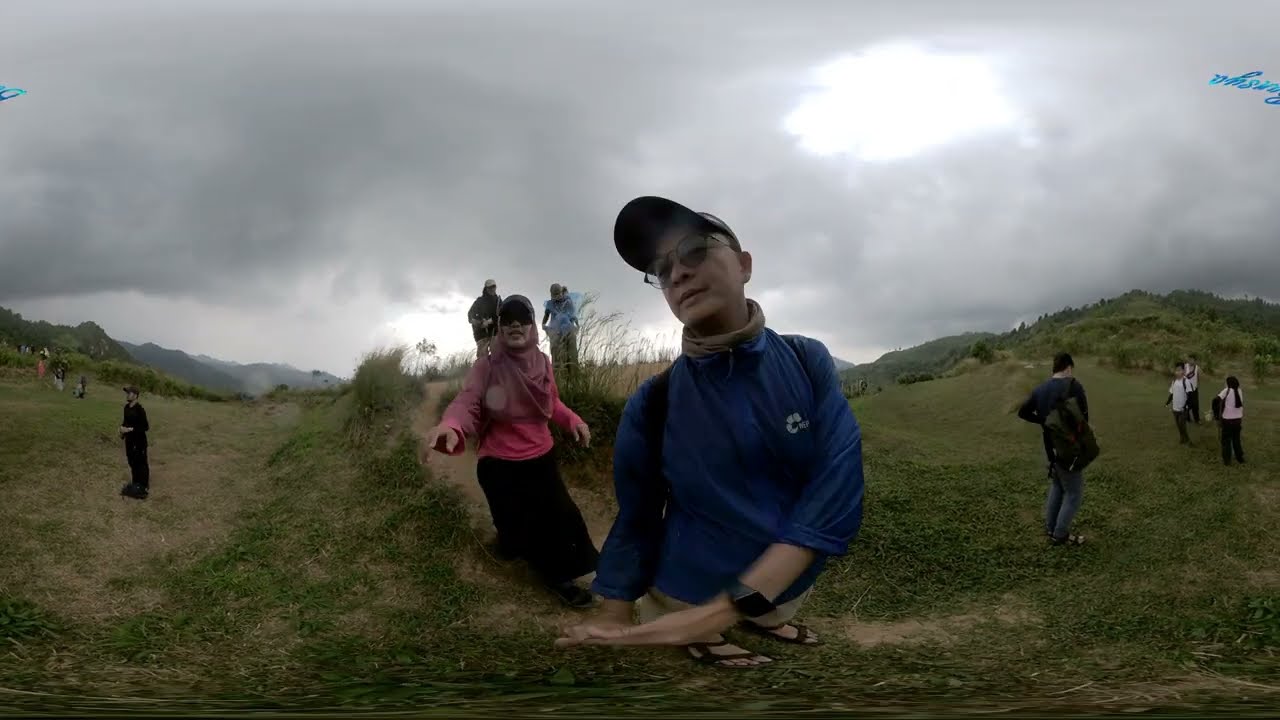This photograph captures a group of people enjoying a hike in a hilly, slightly green field under a very cloudy sky with minimal sunlight peeking through. The focal point is a young man standing at the front, wearing a blue shirt, jeans, a ball cap, glasses, and a jacket, with a watch on his wrist. Next to him is a woman in hiking gear, dressed in a pink shirt and a hat, also sporting a backpack. The ground around them is a mix of light green, somewhat dead grass and scattered dirt piles. 

In the background, there is a mix of other people: a woman in a hijab directly behind the woman in blue, a man in jeans and sneakers to the right, and several others in white shirts spread out in the distance. The backdrop includes rolling hills and large, grayish-blue mountains. The mood is casual and relaxed, with people seemingly enjoying the outdoor scenery and exercise despite the ominous, cloudy skies.